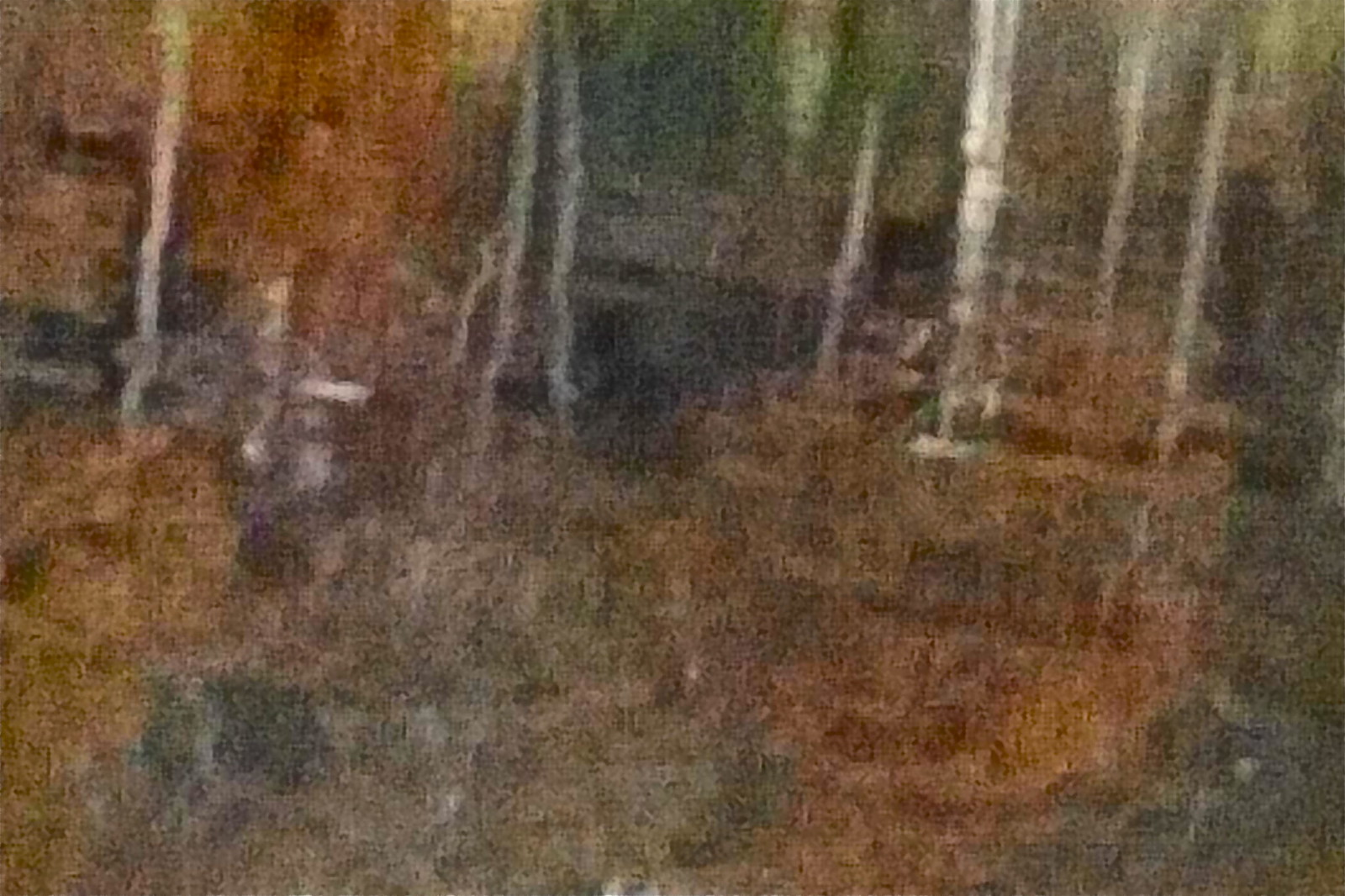A highly abstract and distorted image, reminiscent of a blurred and pixelated oil painting, likely a result of modifications through resizing and filtering during uploading. The scene appears to depict a wooded area with eight slender, white birch tree trunks standing amidst a backdrop of varying shades of green, hinting at a dense forest. The overall composition is characterized by its extreme lack of focus, evoking an almost dreamlike or impressionistic quality.